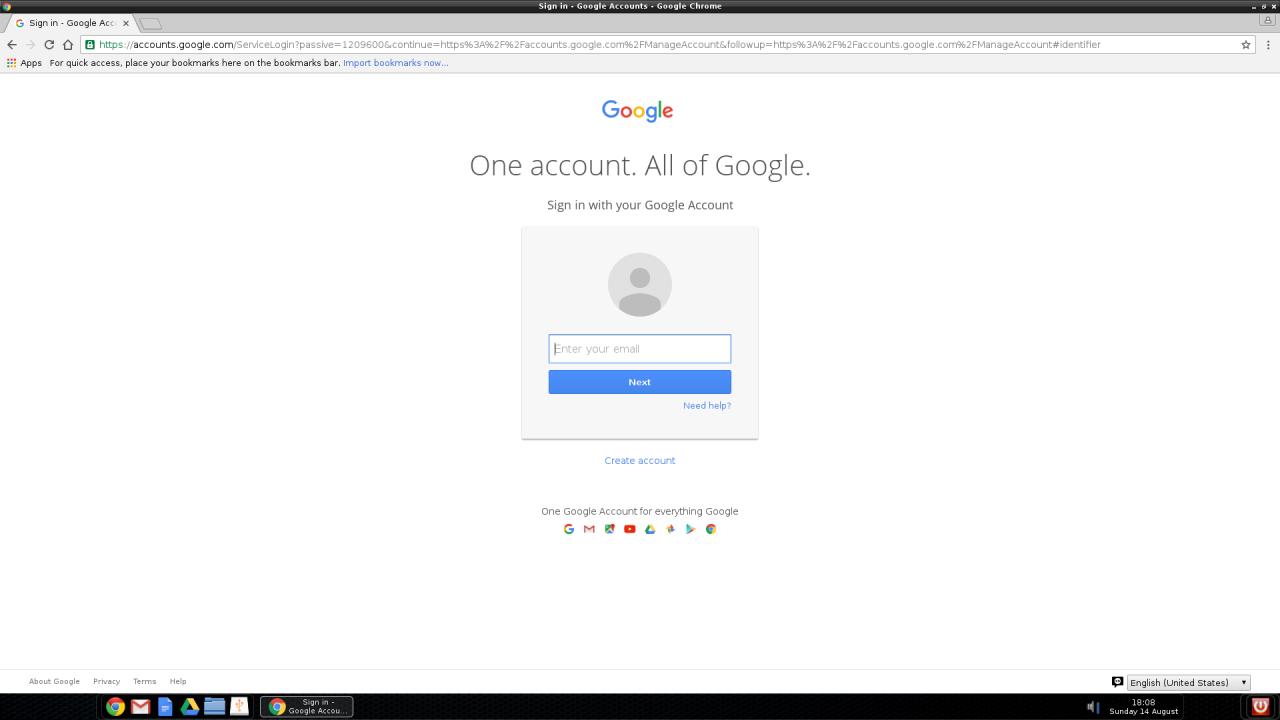The image displays a detailed Google sign-in page against a white background. At the top, a thin black bar features extremely small white text. Below it, there's a grey area showcasing the Google "G" logo, a "Sign in" prompt, a left arrow, a home button, a long search bar ending with a star icon, and a blue line with small text.

In the center, the colorful Google logo (blue, red, yellow, and green) stands out with the phrase "One account. All of Google" below it, instructing users to sign in with their Google account. A blue button beside a circular icon depicting a person's silhouette reads "Next," with fine print beneath it. 

Towards the bottom, assorted Google service icons are displayed. Just above the bottom edge, small text precedes a tiny blue box resembling a search field, accompanied by a small black square with a down arrow on the right side.

Finally, a black box at the bottom section includes various elements: "Your Google," a mail icon, a blue triangle, another blue box, a white box, and a circle filled with Google colors. To the right, there's additional white text and a small red box.

The entire composition appears meticulously structured, offering a comprehensive overview of the application's sign-in interface.